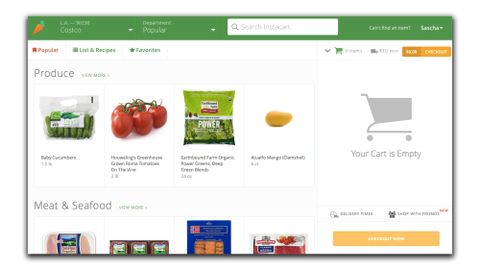A detailed caption for the image could be:

"We are viewing a web page of an online grocery shopping site. The website has a clean, white background with a prominent green banner running across the top. On the left-hand side of the banner, there's an illustration of an orange carrot with vibrant green leaves. 

The page has three tabs, and we are currently on the 'Most Popular' tab within the 'Produce' section. Displayed prominently are fresh red tomatoes, a bag of crisp lettuce, and what appears to be a potato. 

On the right side of the screen, there's a gray icon of a shopping cart indicating that the cart is currently empty. 

Further down, it appears we've accidentally scrolled into the 'Meat and Seafood' section, revealing various items such as a box of shrimp, three packages of ground beef, ham, and bacon towards the bottom of the page."